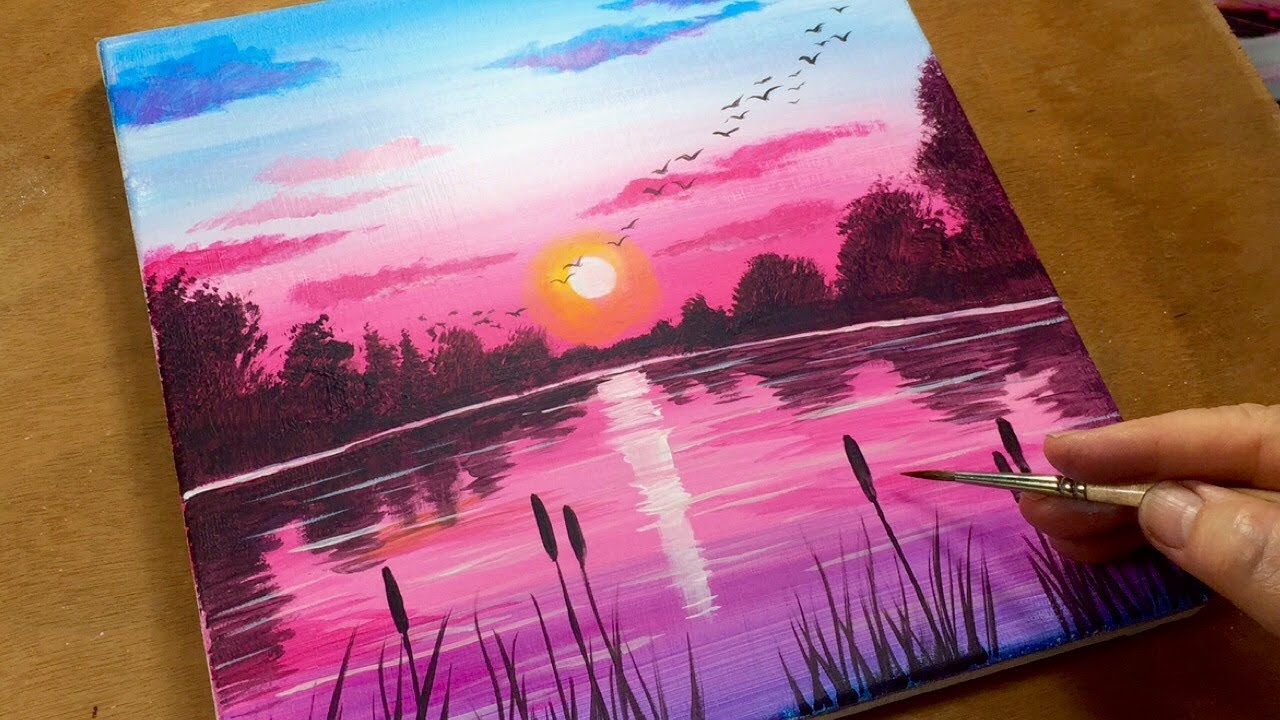In the image, we see a detailed painting set on a brown platform, vividly illustrating a serene sunset scene over a body of water. The painting is dominated by shades of pink and purple, with the sky transitioning from blue at the top to a rich blend of pink and purple near the horizon. The sun is setting at the horizon, casting a beautiful reflection on the water below, which paints the water in similar hues of pink and purple. On either side of the painting, trees also reflecting these colors converge at the center at the horizon. A flock of birds flies across the sky, adding life to the tranquil scene. Closest to the viewer, we observe water plants with their stalks protruding above the water surface, along with the detailed hand of the painter holding a thin paintbrush. The painter’s fingernails are slightly open, which adds a sense of realism and intimacy to the image. This painting captures the picturesque moment of a sunset by the water, framed by nature in beautiful tones.